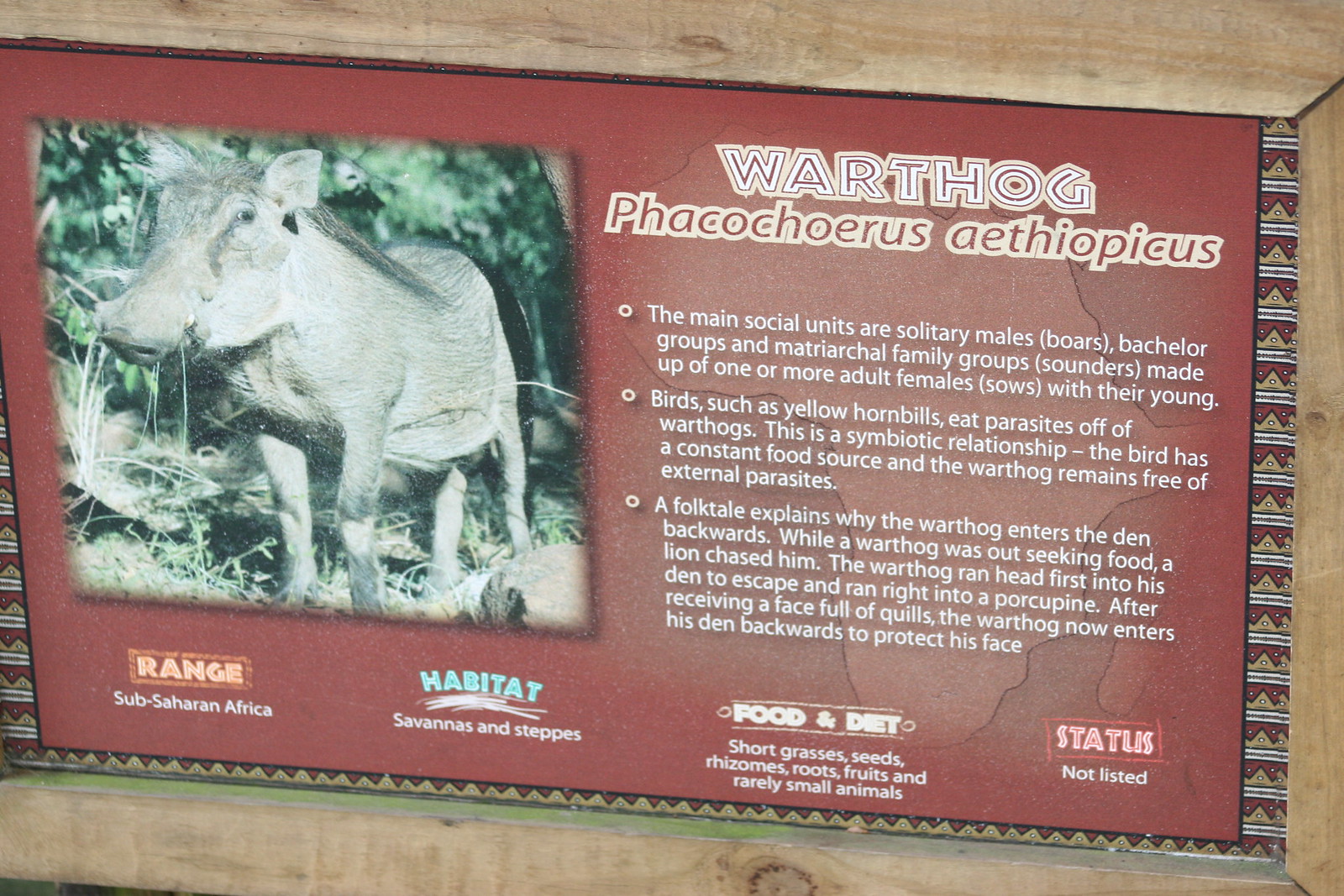The image features an educational display about the warthog against a reddish-brown background. At the top, the word "Warthog" is prominently displayed in white text, accompanied by a picture of the animal on the left. The warthog's scientific name, *Phacocorys aethiopychus*, is also provided. The display is organized into various sections detailing the warthog's characteristics and life:

1. **Range**: Sub-Saharan Africa
2. **Habitat**: Savannas and steppes
3. **Food and Diet**: Short grasses, seeds, rhizomes, roots, fruits, and rarely small animals
4. **Status**: Not listed

Additionally, it mentions the warthog's social structure, noting that the main social units include solitary males (boars), bachelor groups, and matriarchal family groups (sows and their young). There is also an explanation of the symbiotic relationship between warthogs and birds like yellow hornbills, which eat parasites off the warthogs, benefiting both species. The display includes several sponsors at the bottom.